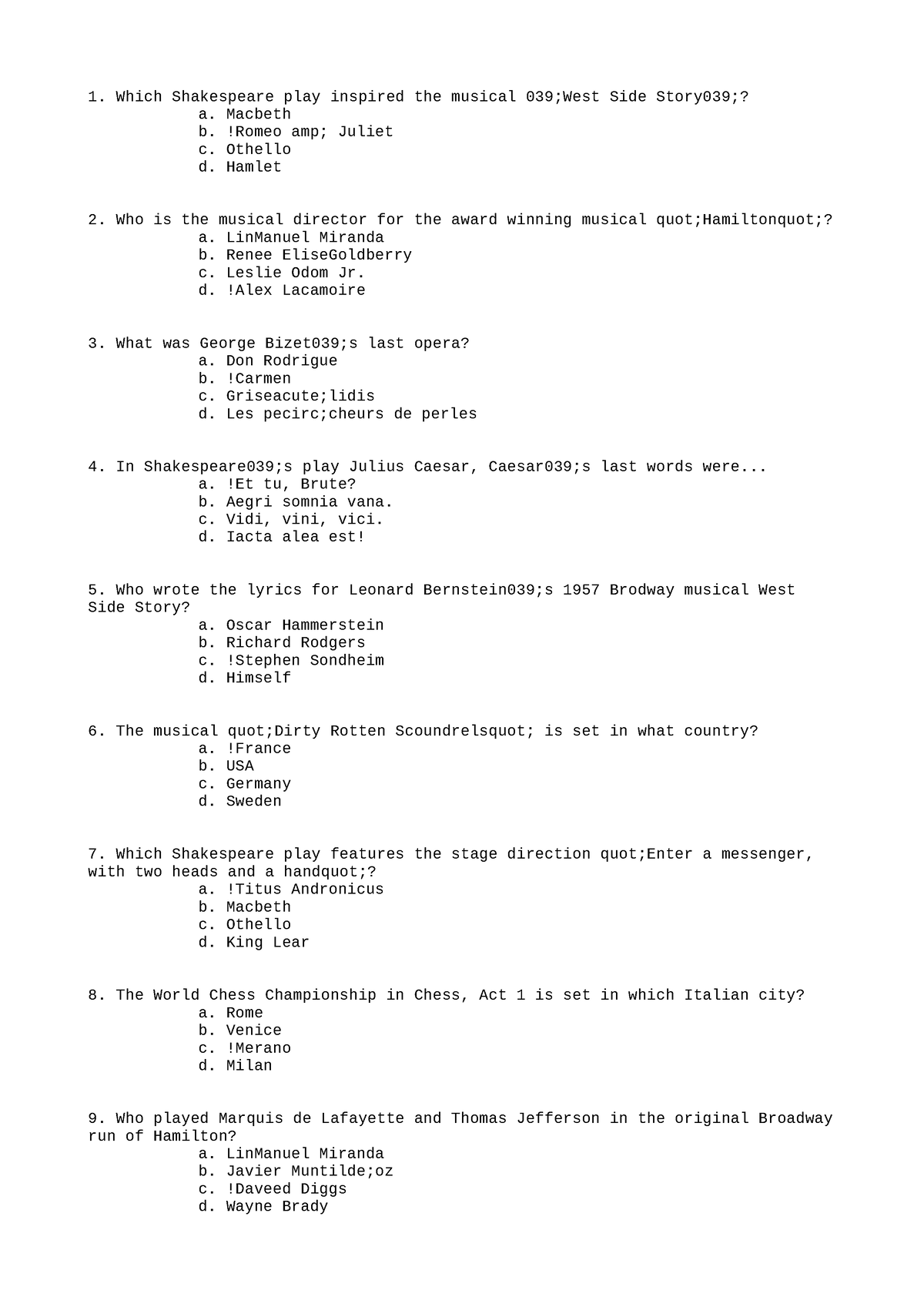### Detailed Caption for the Document Image

The image is a clean, white background document featuring black font, arranged in a quiz format. The document appears to be a multiple-choice test with a total of nine questions, each offering four answer options labeled A through D. However, the correct answers are not indicated.

1. **Question 1:** "Which Shakespeare play inspired the musical *West Side Story*?" 
   - **Options:** 
     - A. Macbeth
     - B. Romeo and Juliet
     - C. Othello
     - D. Hamlet

2. **Question 2:** "Who is the musical director for the award-winning musical *Hamilton*?"
   - **Options:** 
     - A. Lin-Manuel Miranda
     - B. Renée Elise Goldsberry
     - C. Leslie Odom Jr.
     - D. Alex Lacamoire

3. **Question 3:** "What was George Bizet's last opera?"
   - **Options:** 
     - A. Don Rodrigue
     - B. Carmen
     - C. L'Arlésienne
     - D. Les Pêcheurs de Perles

4. **Question 4:** "In Shakespeare's play *Julius Caesar*, Caesar's last words were?"
   - **Options:** 
     - A. Et tu, Brute?
     - B. Egas summa vena
     - C. Veni, vidi, vici
     - D. Iacta alea est

5. **Question 5:** "Who wrote the lyrics for Leonard Bernstein’s 1957 Broadway musical *West Side Story*?"
   - **Options:**
     - A. Oscar Hammerstein II
     - B. Richard Rodgers
     - C. Stephen Sondheim
     - D. Leonard Bernstein himself

6. **Question 6:** "The musical *Dirty Rotten Scoundrels* is set in which country?"
   - **Options:**
     - A. France
     - B. USA
     - C. Germany
     - D. Sweden

7. **Question 7:** "Which Shakespeare play features the stage direction, 'Enter a Messenger with two heads'?"
   - **Options:**
     - A. Titus Andronicus
     - B. Macbeth
     - C. Othello
     - D. King Lear

8. **Question 8:** "The *World Chess Championship* Act One is set in which Italian city?"
   - **Options:**
     - A. Rome
     - B. Venice
     - C. Merano
     - D. Milan

9. **Question 9:** "Who played Marquis de Lafayette and Thomas Jefferson in the original Broadway run of *Hamilton*?"
   - **Options:**
     - A. Lin-Manuel Miranda
     - B. Javier Muñoz
     - C. Daveed Diggs
     - D. Wayne Brady

The questions cover a range of topics related to musicals and Shakespearean plays, reflecting a focus on theatre and literary knowledge. The document seems designed for an audience familiar with classic literature and musical theatre.